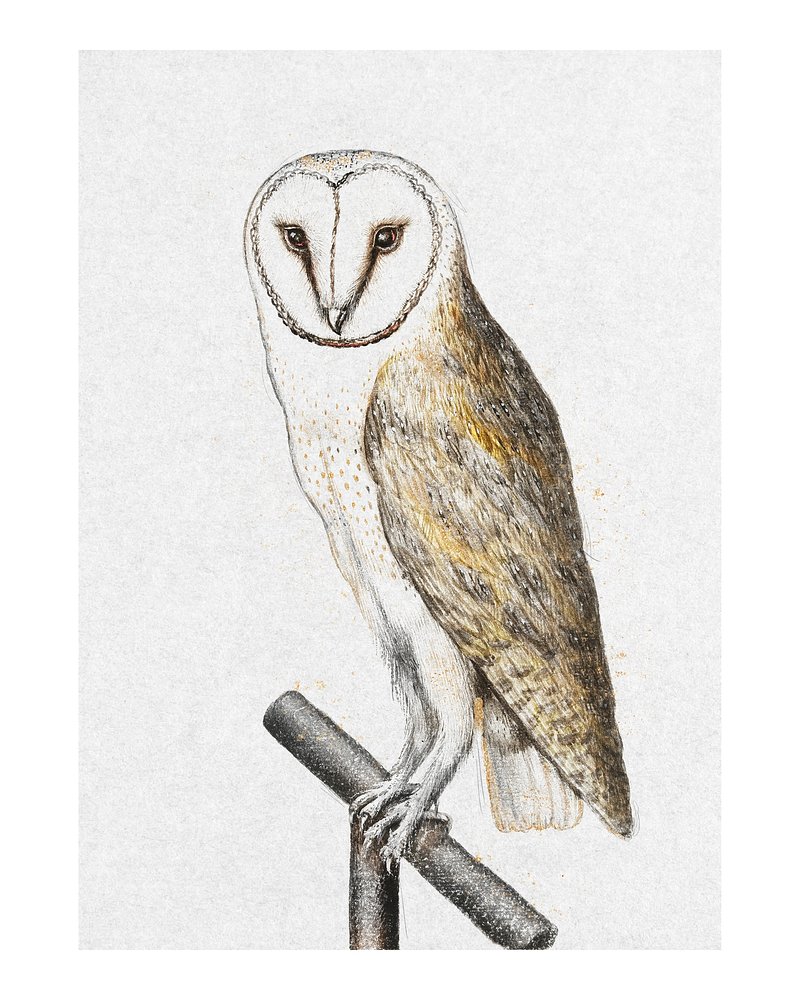This artistic depiction of a barn owl presents a richly detailed and textured illustration, possibly created with colored pencils. The owl, positioned centrally against a light grayish background, stands on a dark brown, wooden perch designed for birds. The owl itself showcases a harmonious blend of colors: its chest is predominantly white adorned with fine brown dots, while its back features an array of light brown feathers with interspersed darker brown and whiter patches. The owl's striking face, turned toward the viewer, is framed by white feathers around its eyes, which are a deep dark brown. Its beak and talons have a yellowish hue, adding to the realistic portrayal. The absence of any signature or text emphasizes the image's focus on the detailed and lifelike representation of the owl, reminiscent of vintage scientific illustrations meant to showcase the bird's appearance and size.